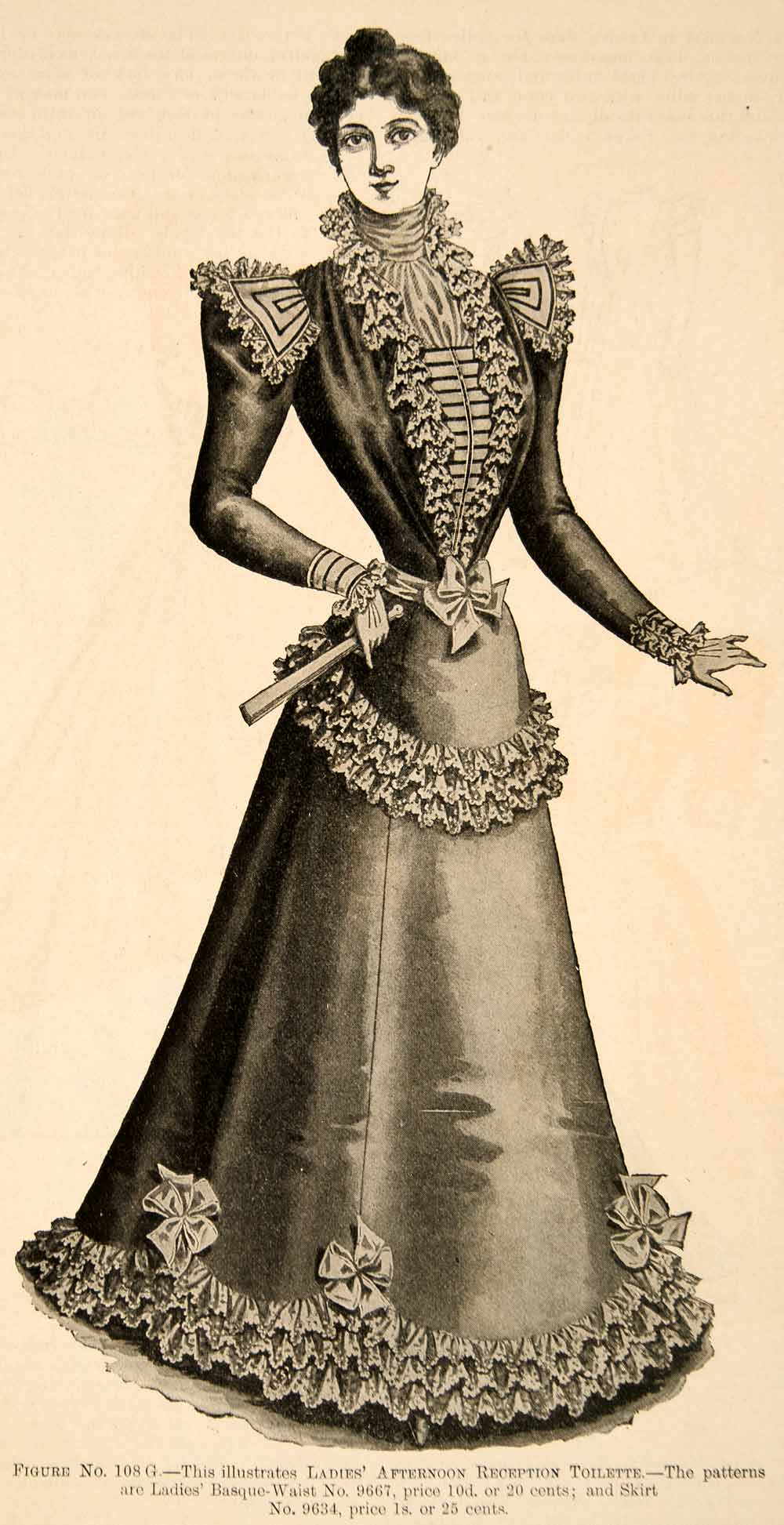The image is an intricate black and white artwork, likely an illustration from a women's fashion magazine dating back to the late 1800s. The drawing is set against a cream-colored or yellowed background, suggestive of an aged newspaper page. It features a woman wearing an elaborate Victorian dress, characterized by a highly cinched waist that accentuates the A-line skirt, which cascades down to the floor, concealing her shoes. Her dark hair is styled in a bun at the top center of her head, and she has a long, slender nose, a slight smirk, and open eyes.

The dress is highly detailed: the blouse has long sleeves with ruffled edges and a frilly front that extends down to her midsection. An underblouse with a ruched top turtleneck peeks out from underneath the main blouse. Large, square shoulder pads extend to the sides, mirroring the ruffled style of the centerpiece. Around her cinched waist, tied with a bow, the skirt flares out, adorned with multiple layers of ruffles and intermittent tied ribbons, creating a tiered effect down to the floor. 

She holds a fan in her right hand while her left hand is extended with an open palm. Text at the bottom reads figure number 108G and describes the patterns: lady basque waist number 9667, priced either 10 cents or 20 cents, and skirt number 9634, priced 1 cent or 25 cents.